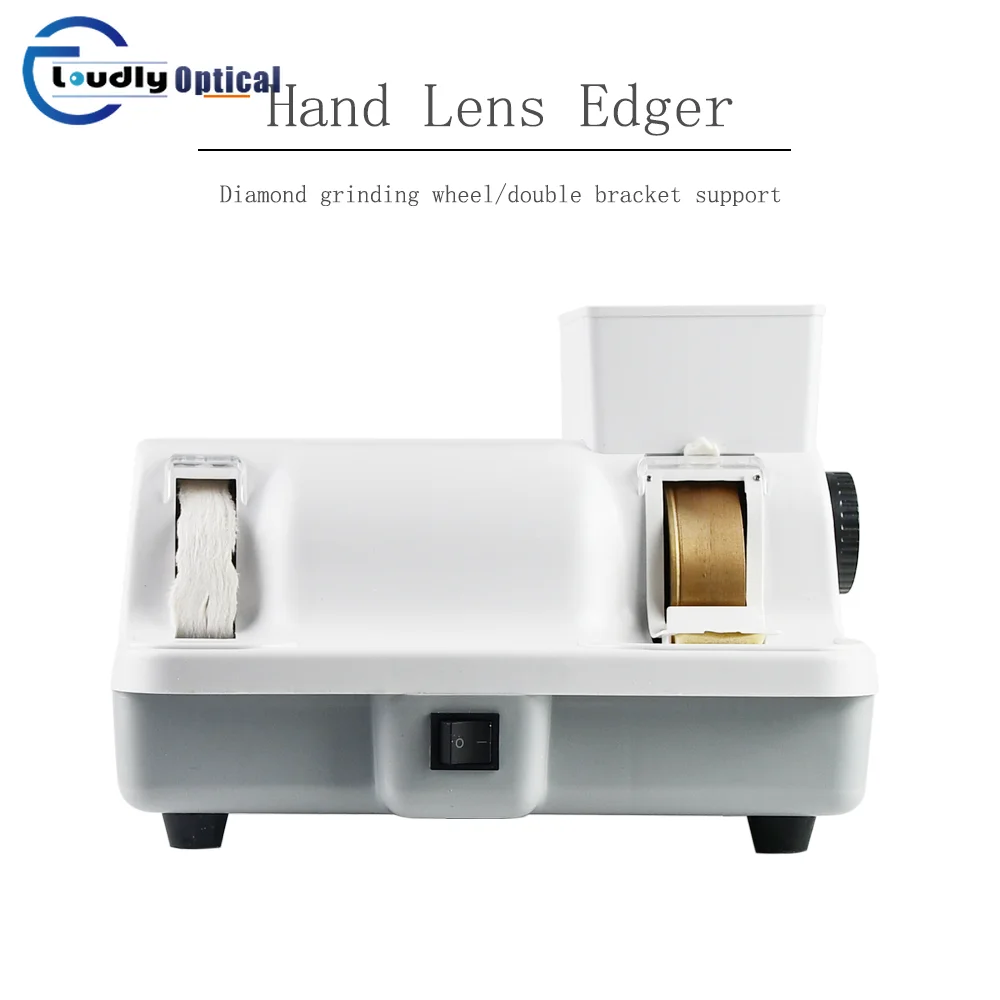This image showcases a hand lens edger, a piece of equipment from Loudly Optical. The company logo, along with the product name, "Hand Lens Edger," is prominently displayed in the top left corner of the image, accompanied by the text "Diamond Grinding Wheel / Double Bracket Support," underlined for emphasis. The edger itself is a white, boxy unit with sturdy black feet for stability, designed to be placed on a tabletop. On the front of the unit, there is a black power button in the off position, which controls the machine. The right side features a black plastic spin wheel, potentially for adjusting the speed or tension of the grinding wheel. The front of the machine showcases a prominently labeled diamond grinding wheel, emphasizing its dual functionality with the double bracket support. This setup suggests that the machine is used for grinding and polishing the edges of lenses, making it a vital tool in the optical industry. The simple and robust design highlights its practical application, likely for promotional purposes.